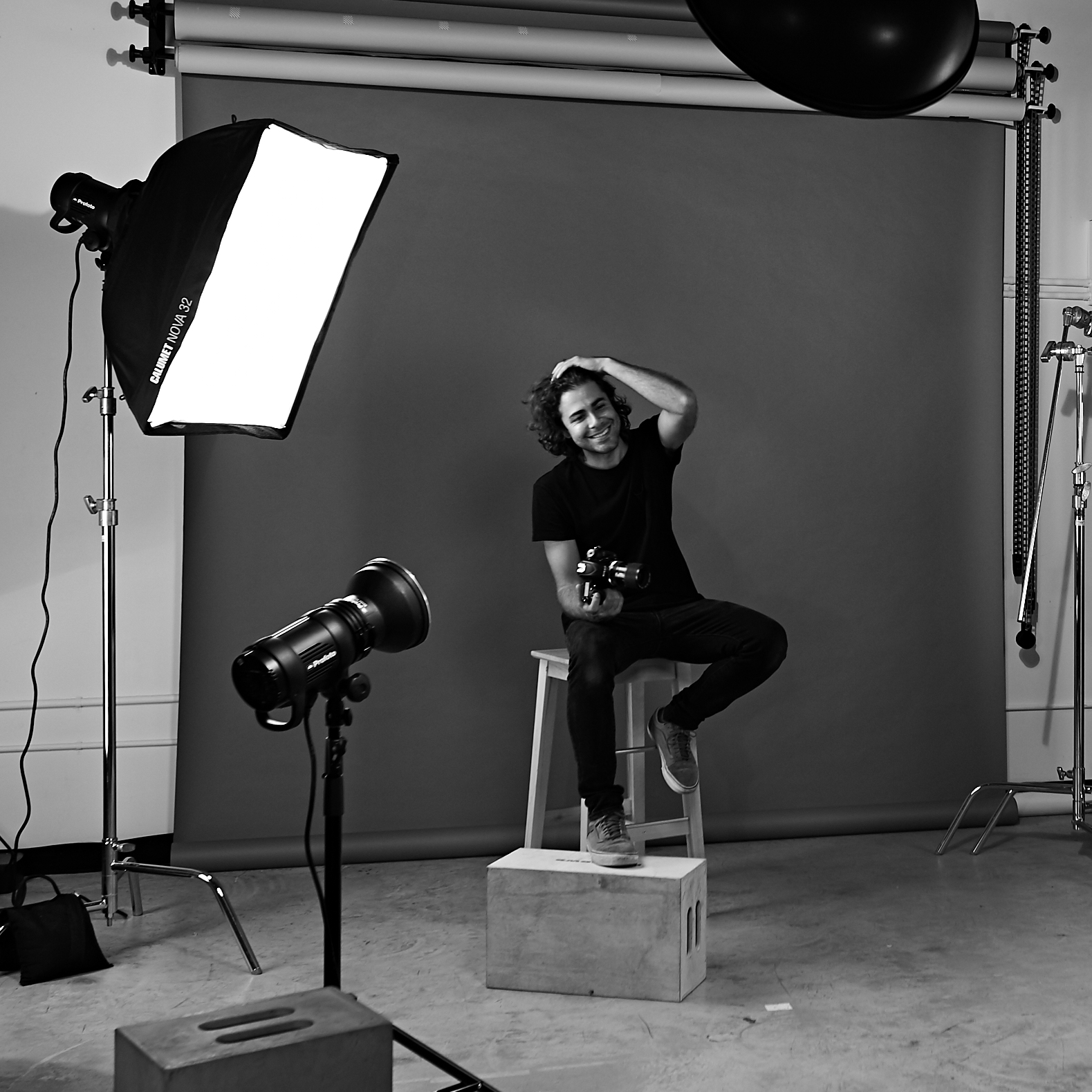This black and white photograph captures a behind-the-scenes moment of a photo shoot. At the center, sitting on a wooden stool, is a young man with long, curly black hair that reaches his shoulders. He is dressed in a black t-shirt, dark jeans, and sneakers. His left foot is propped up on a wooden block while his right leg rests on the ground. The man is smiling and looking slightly down and to the right, with his left hand running through his hair and his right hand holding a black camera.

Behind him, a dark-colored backdrop is pulled down, revealing its roll-up mechanism at the top. Bright photography lights illuminate the scene; a large square light marked "Nova 32" shines from the left side, while a smaller light in the front-left corner casts additional illumination. The floor appears to be made of concrete, adding to the utilitarian atmosphere. A tripod is partially visible on the right side of the image, contributing to the sense of an active photo studio environment. Another wooden crate, similar to the one under the man's foot, is also present in the scene.